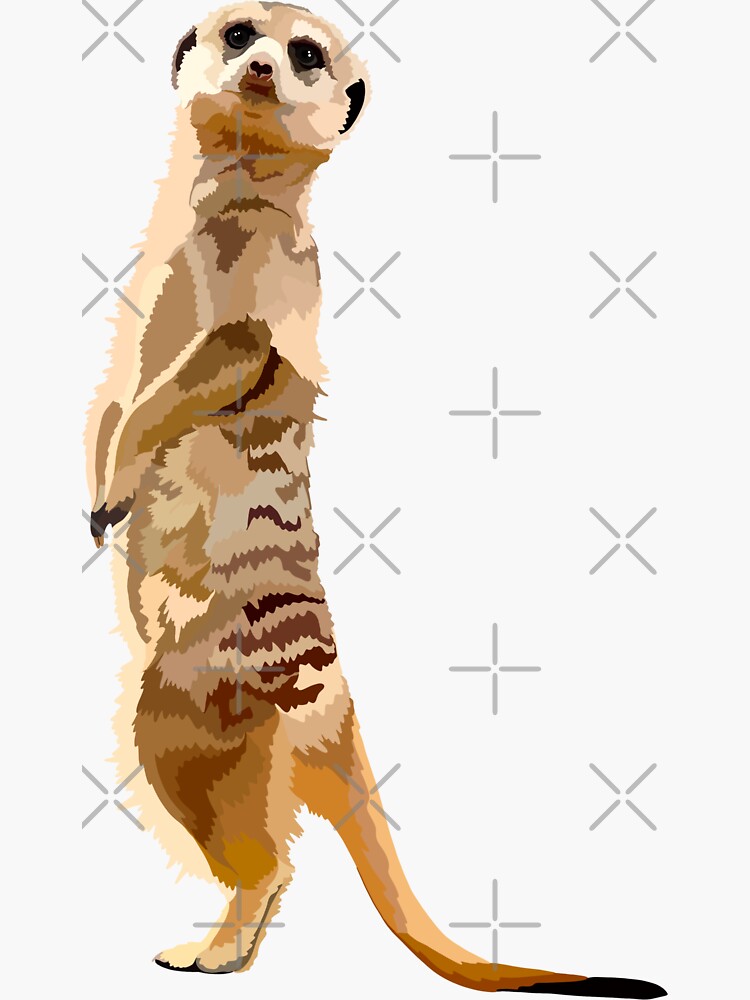This digital illustration features a detailed depiction of a meerkat standing on its hind legs in a classic upright stance. The meerkat, with its tan, cream, and beige body accented by light, dark brown, and gray-brown hues, is positioned on the left side of the frame, its profile facing sideways while its head looks directly at the viewer. Distinctive large black eyes, a small brown nose, and tiny black ears characterize its expressive face. Its arms rest in front of its belly, and its tail, predominantly beige with a black tip and brown accents, trails behind it on the ground. The background is a soft light gray, and the image is overlaid with a watermark consisting of dark gray X's and plus signs, giving it a textured look.